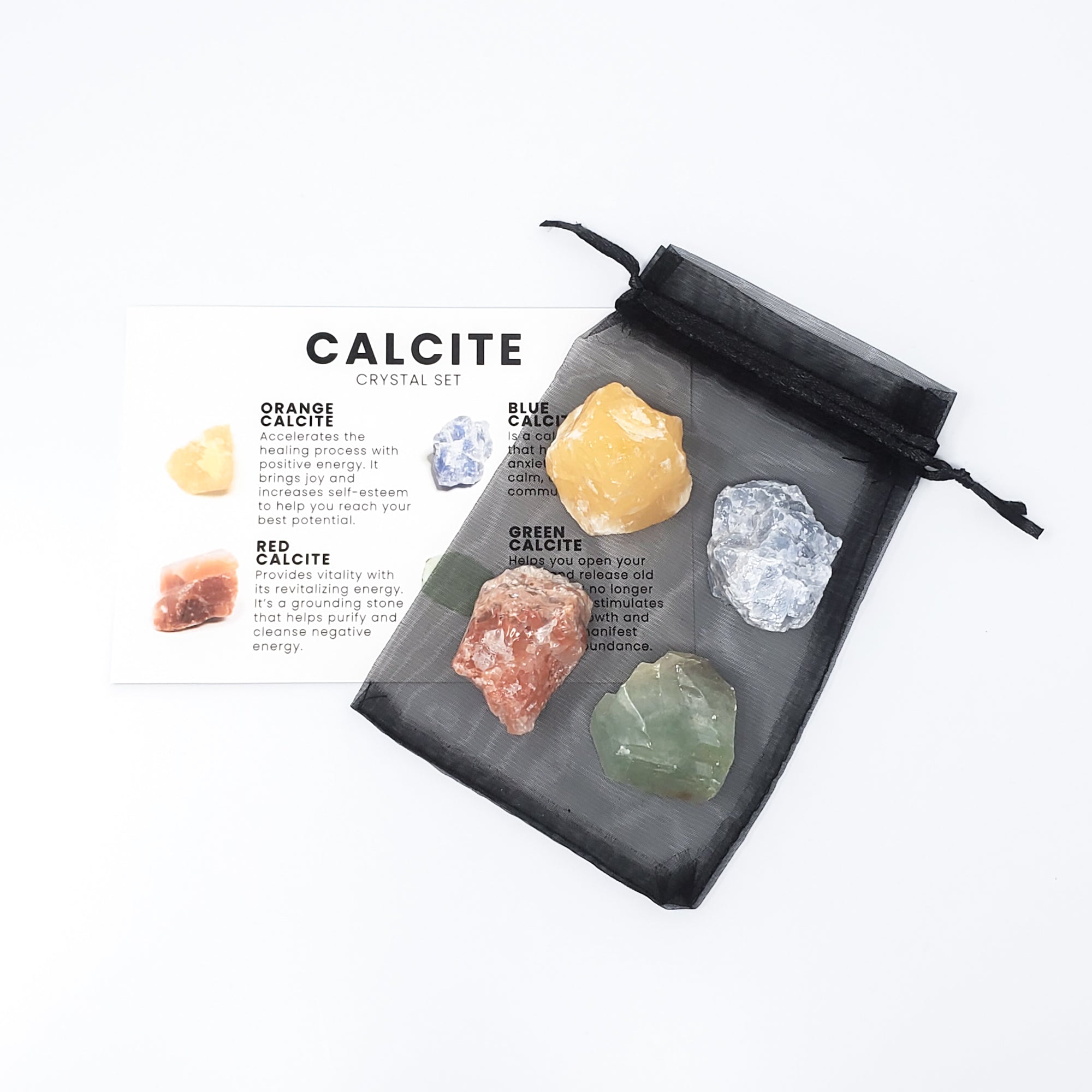The image is set against a light blue or almost white background, featuring a central informational white card partially obscured by a black mesh bag, which is angled from the bottom left to the top right. The bag has a black top with a drawstring closure. The white card, visible on the left side, prominently displays the title "Calcite" in large black letters with "Crystal Set" in smaller gray letters beneath it. On the left side of the card, there are descriptive lines next to images of stones. It lists "Orange Calcite" at the top, with its description indicating properties such as accelerating the healing process and bringing joy. Below that is "Red Calcite," described as providing vitality and grounding. On the right side, partially visible through the mesh bag, the card mentions "Blue Calcite," next to a blue stone, and "Green Calcite," next to a green stone. The black mesh bag contains four crystals arranged in rows of two: an orange stone on the top left, a blue stone on the top right, a red stone on the bottom left, and a green stone on the bottom right. The bag is see-through, allowing identification of each calcite stone corresponding to the descriptions on the card.